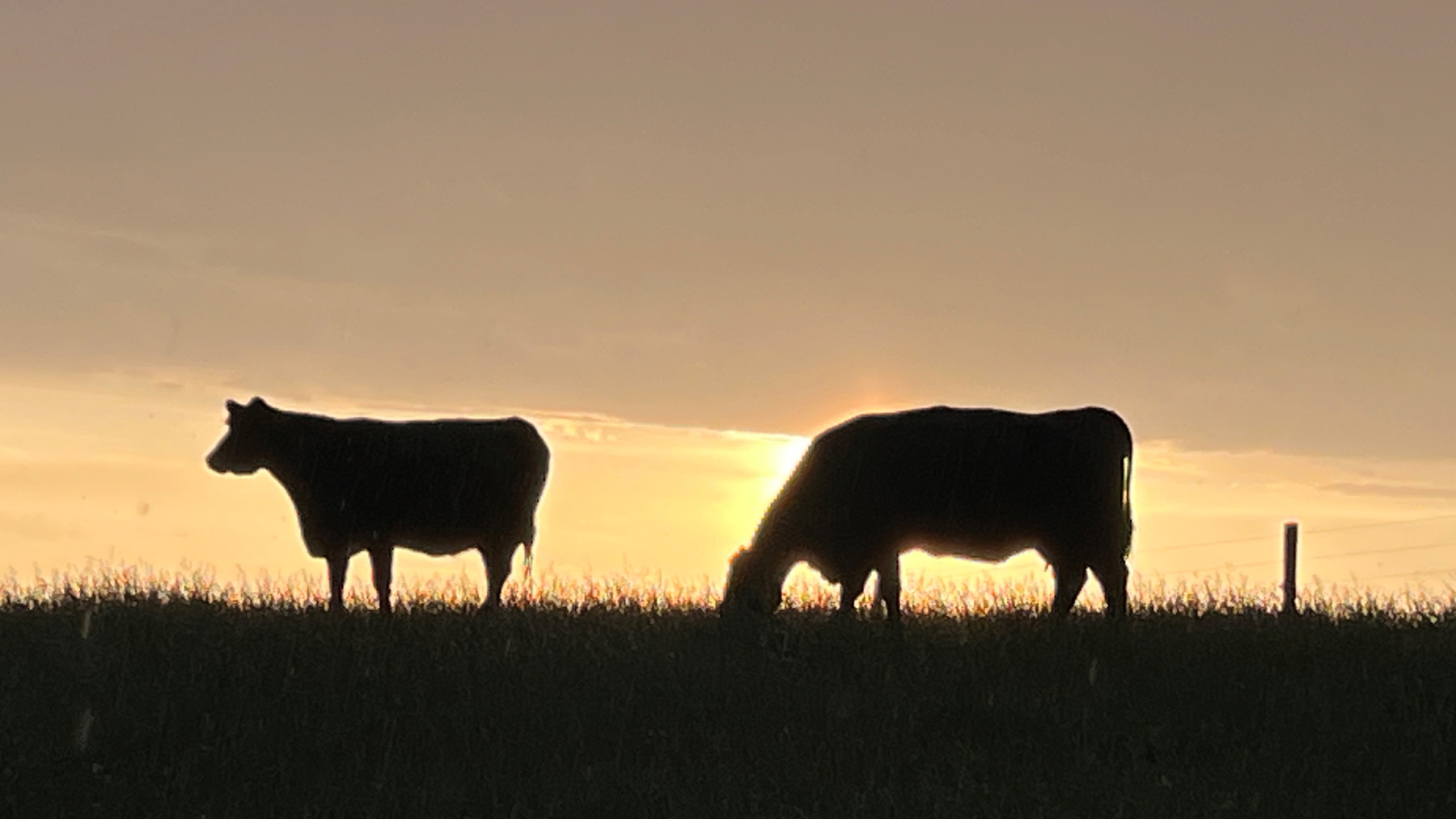The image depicts a serene and still scene at dusk, showcasing two cows grazing in a field with an orange-tinted sky due to the low sunlight either from the rising or setting sun. One cow is engrossed in eating grass with its head down, while the other stands alert with its head up, surveying the surroundings. Both cows are silhouetted against the horizon, appearing as dark figures due to the backlighting from the sun. The sky above them is darker gray, suggesting the impending night or storm clouds. A wooden post fence with wire lines can be seen in the background, enclosing the field and adding to the pastoral setting. The cows and fence create a harmonious rural scene, capturing a moment of quiet tranquility.